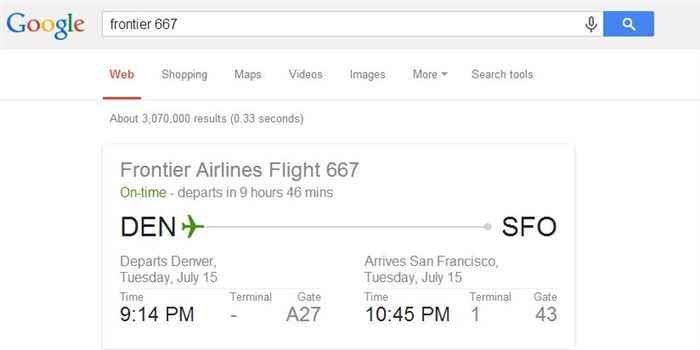The image showcases a detailed flight information panel for a Frontier Airlines flight. The panel itself is a clean, white rectangular box adorned with grey and black text, alongside some minimal color highlights for emphasis. The text primarily informs that the flight is "on time" and is scheduled to depart in 9 hours and 46 minutes from Denver International Airport (DEN) to San Francisco International Airport (SFO). 

Specifically, the departure is set for Tuesday, July 15th at 9:14 PM from gate A27 in Denver, with an arrival in San Francisco at terminal 1, gate 43 at approximately 10:45 PM on the same day. The word "on time" and a small airplane icon are both accented in green, standing out against the otherwise monochromatic palette of the design. Overall, the presentation is straightforward and functional, aimed at efficiently conveying the essential flight details without any unnecessary embellishments.